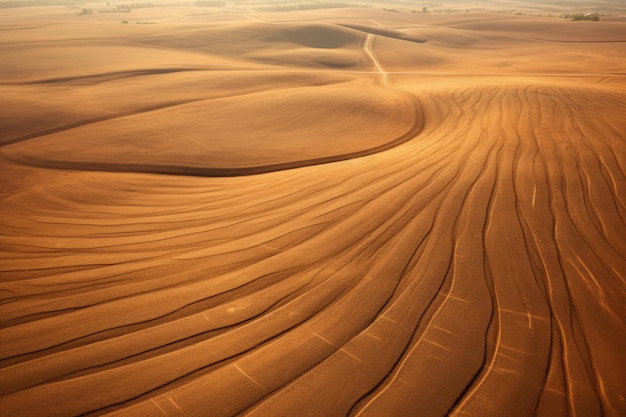This image showcases a vast desert landscape dominated by orange and light brown sands stretching endlessly across the frame. The desert floor is divided into two distinct sections. On the right-hand side, the sand displays intricate patterns, resembling rows of curves or swirls, perhaps created by a rake or some natural force. These lines weave a textured tapestry that contrasts sharply with the left-hand side, where the sand remains untouched, smooth, and pristine, featuring minor dips and valleys. The sand transitions from a deep, dark tan to a lighter brown, creating a sense of depth and movement. In the middle of the photo, a thin line of darker brown sand extends into the distance, guiding the eye toward the far background. Here, subtle rolling hills are visible, some with hints of gray, and in the furthest background, there seems to be either the outline of a distant city or a patch of green vegetation, suggesting the presence of an oasis. The image is clear and modern, capturing the serene yet intricate beauty of the desert landscape in high detail.